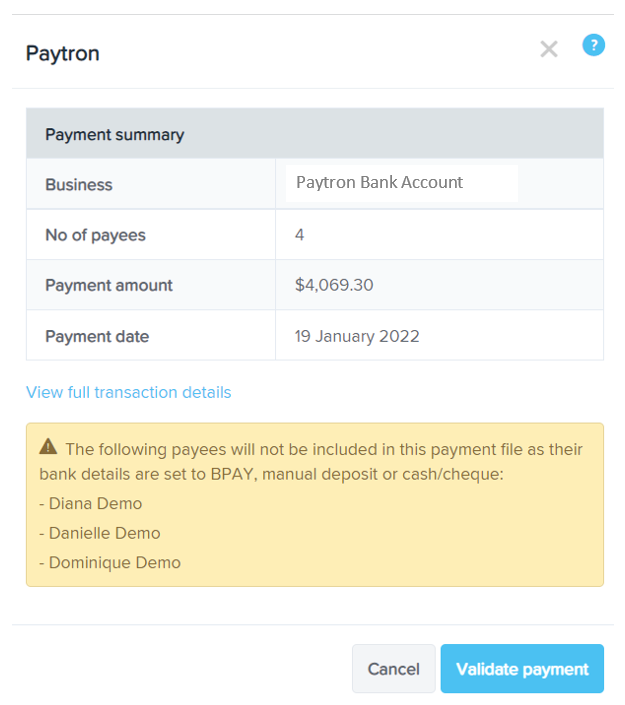The image appears to show a web page related to financial transactions. At the top left corner, a logo or title reads "Patron." The page is otherwise mostly blank in the middle. Across the top are navigation elements, including an "X" for closing the page and a blue circle containing a question mark, likely linking to a help section.

Underneath these navigation elements, a section titled "Payment Summary" is positioned on the left side of the page. This section begins with a dark gray bar labeled "Payment Summary." Below this bar, sequentially from top to bottom and left to right, the following details are listed:

1. Business: "Patron Bank Account"
2. Number of Payees: "4"
3. Payment Amount: "$4,069.30"
4. Payment Date: "19 January 2022"
5. A blue hyperlink labeled "View Full Transaction Details"

Further down the page, a large yellow box with a warning icon—a triangle containing an exclamation point—warns users: "The following payees will not be included in this payment file as their bank details are set to BPay, manual deposit, or cash/check." Below this warning are the names of individuals not included in the payment:
- Diana Demo
- Daniel Demo
- Dominique Demo

At the bottom right corner of the page, there are two clickable button options: "Cancel" (in gray) and "Validate Payment" (in blue).

This detailed caption should provide a precise and comprehensive understanding of the web page's content and structure.